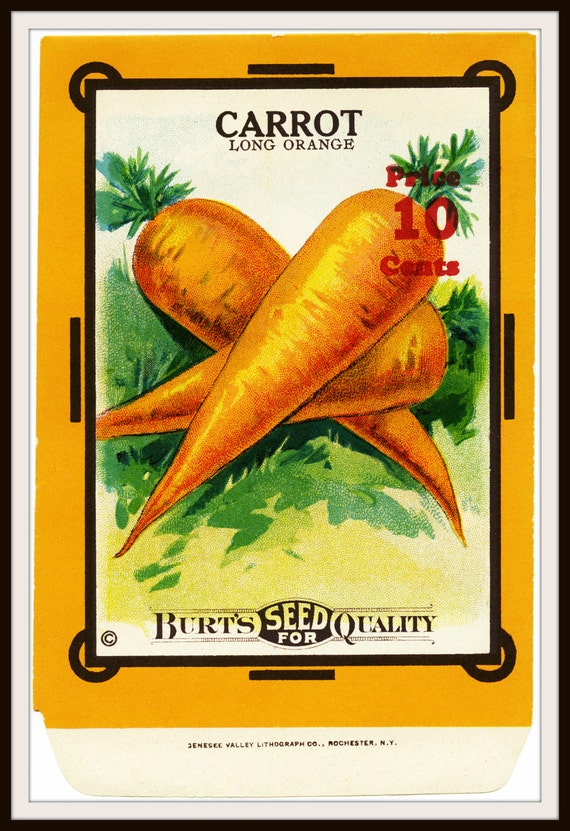The image depicts a vibrant seed packet for carrots from Burt's Seed, noted for its quality. At the top of the packet, "Carrot" is prominently displayed in large print with "Long Orange" beneath it, and to the right, it indicates a price of 10 cents. Below the text, there is a watercolor illustration of three unpeeled, bright orange carrots with green tops, crisscrossing each other. The stems of the carrots are oriented differently: one points to the top left, another to the right, and the topmost carrot points to the top right. These carrots are set against a green, grass-like background, and the image is enclosed in a black square. The package transitions in color from black at the top to white and then to a bright orange at the bottom. At the bottom, the text reads "Burt's Seed for Quality," and further below, it mentions "Genesee Valley Lithograph Company, Rochester, New York."